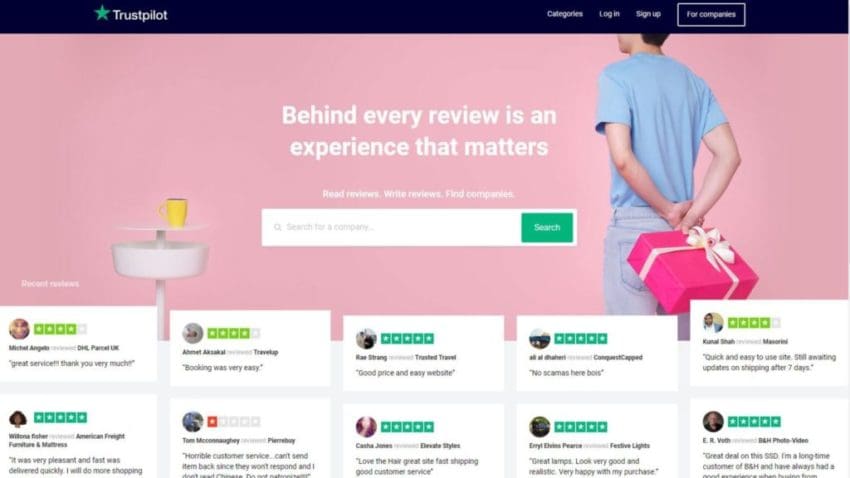The image features a prominent rectangle at the top, which appears to be either a very dark blue or black. Towards the left side of this rectangle, there is a green star next to the text "Trust Pilot". On the right side, there are some indistinct words, along with another smaller rectangle that is outlined in white and has white text inside, which is too small to decipher.

Beneath this, there is a large pink rectangle. On the right side of this pink rectangle stands a man with his hands behind his back, holding a gift. He is dressed in a blue t-shirt and blue jeans. Towards the left of the pink rectangle, there's an object that is difficult to identify, but it appears to resemble a cup placed on top of a white line. Beneath this line, there's a white bowl shape with a line running through or under it.

The pink rectangle also features the text, "Behind every review is an experience that matters", followed by additional text that is too small to read clearly.

Below these elements is a white rectangle. Inside this rectangle, on the left side, there is an icon that looks like a magnifying glass next to more unidentifiable text. On the right side of this white rectangle, there is a green rectangle with the word "Search".

At the bottom of the image, there are ten reviews, each accompanied by stars, although the writing in these reviews is too small to read.